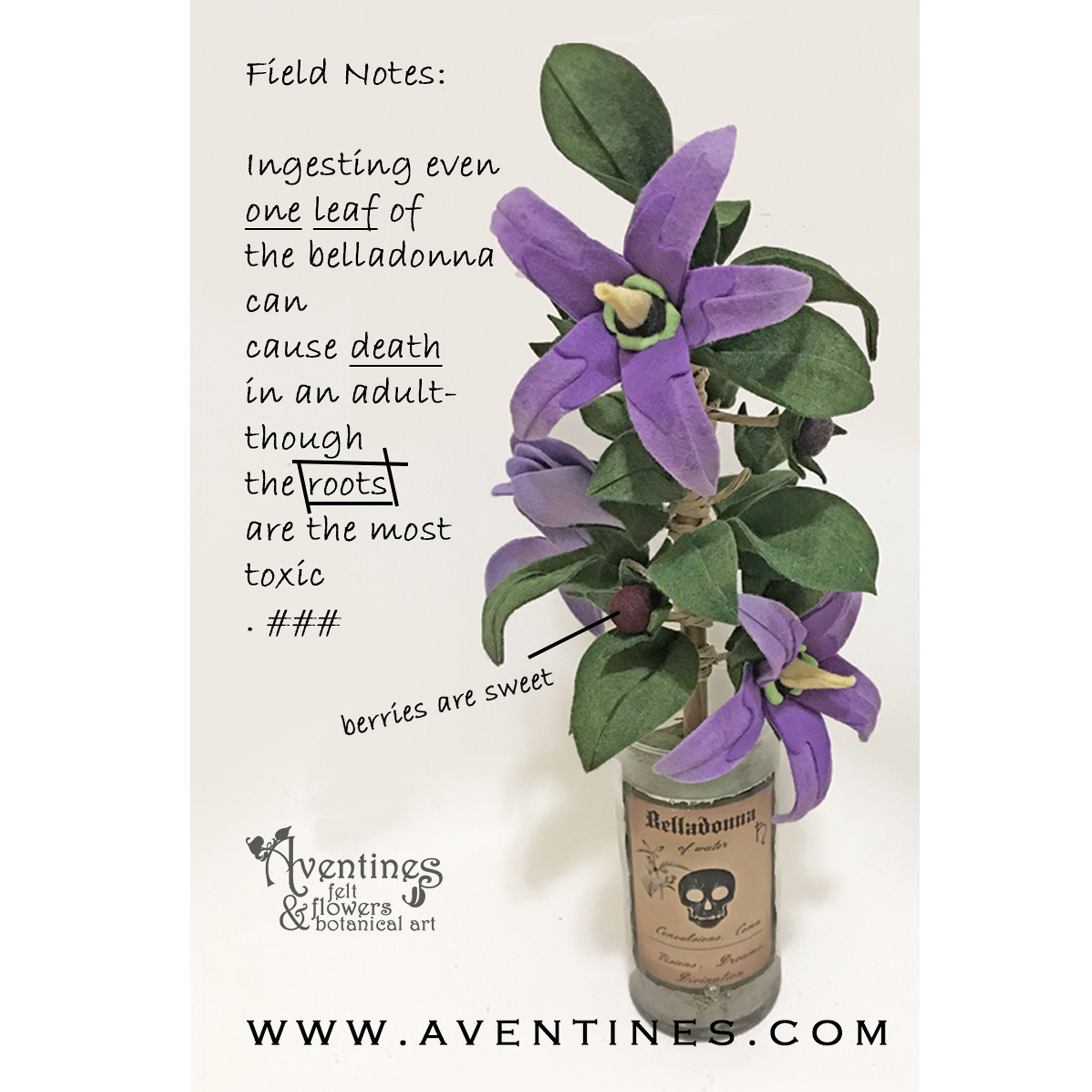This image appears to be an advertisement for Aventines Felt Flowers and Botanical Art, possibly sourced from a magazine or as a dedicated poster. The ad's dimensions are taller than they are wide. The prominent feature of the image is a glass bottle with a pink label bordered in black, prominently marked with the name "Belladonna" and an image of a black skull beneath the text. The bottle contains a botanical plant with green leaves, purple flowers boasting five petals with yellowish-white centers, and some purple berries. 

On the right-hand side of the ad, there is detailed cautionary text under the heading "Field Notes." The text warns: "Ingesting even one leaf of the Belladonna can cause death in an adult, though the roots are the most toxic." Further down, it simply states, "The berries are sweet," with a pointer indicating a berry in the image. Embedded within the design are the words "Aventines Felt Flowers and Botanical Art," and at the very bottom, the website www.aventines.com is displayed in black block lettering.